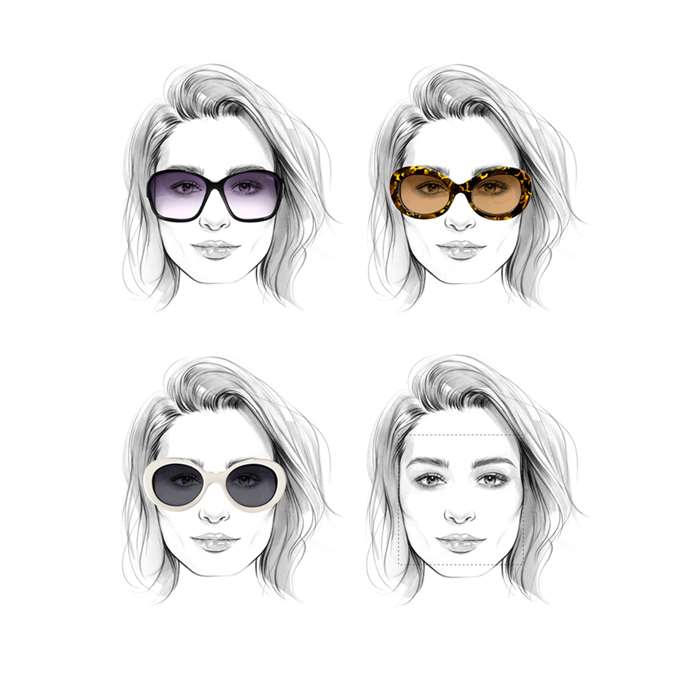The image is an artistic, black-and-white sketch of a young woman in her 20s, depicted four times in a vertically rectangular, borderless format against a white background. Each of the four sections shows her with different eyewear except for one. In the top left, she wears dark-framed sunglasses with purple-tinted lenses through which her eyes are faintly visible. The top right illustration features her in larger brown frames decorated with yellowish metal flecks and brownish lenses. The bottom left section shows her in white-framed sunglasses with smoky gray lenses. The bottom right depiction is of her without glasses but includes a unique dotted box pattern extending from her eyes to her lips. Her blonde hair flows down to her shoulders in all four images.